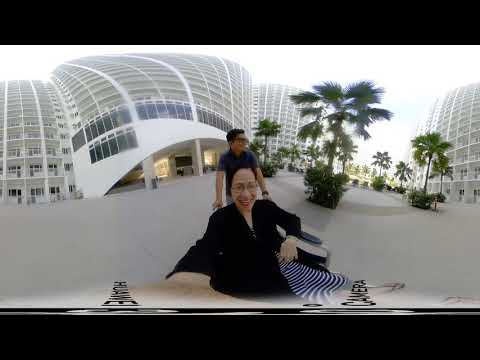In this outdoor scene, a woman with dark hair, wearing glasses, a black jacket, and a black and white dress sits and smiles at the camera. She holds a purse or bag over her left shoulder. Her eyelids are slightly closed, giving her a gentle expression. Behind her stands a man with dark hair and glasses, dressed in a blue shirt, who appears to be possibly pushing her in a wheelchair. They are situated in a spacious courtyard adorned with several large, white, multi-storied buildings featuring numerous windows and balconies. To the right, there are about 10-15 palm trees lined up in large planters, adding a tropical touch to the landscape. The day is slightly overcast with a gray and hazy sky, yet some sunlight filters through, illuminating the scene.